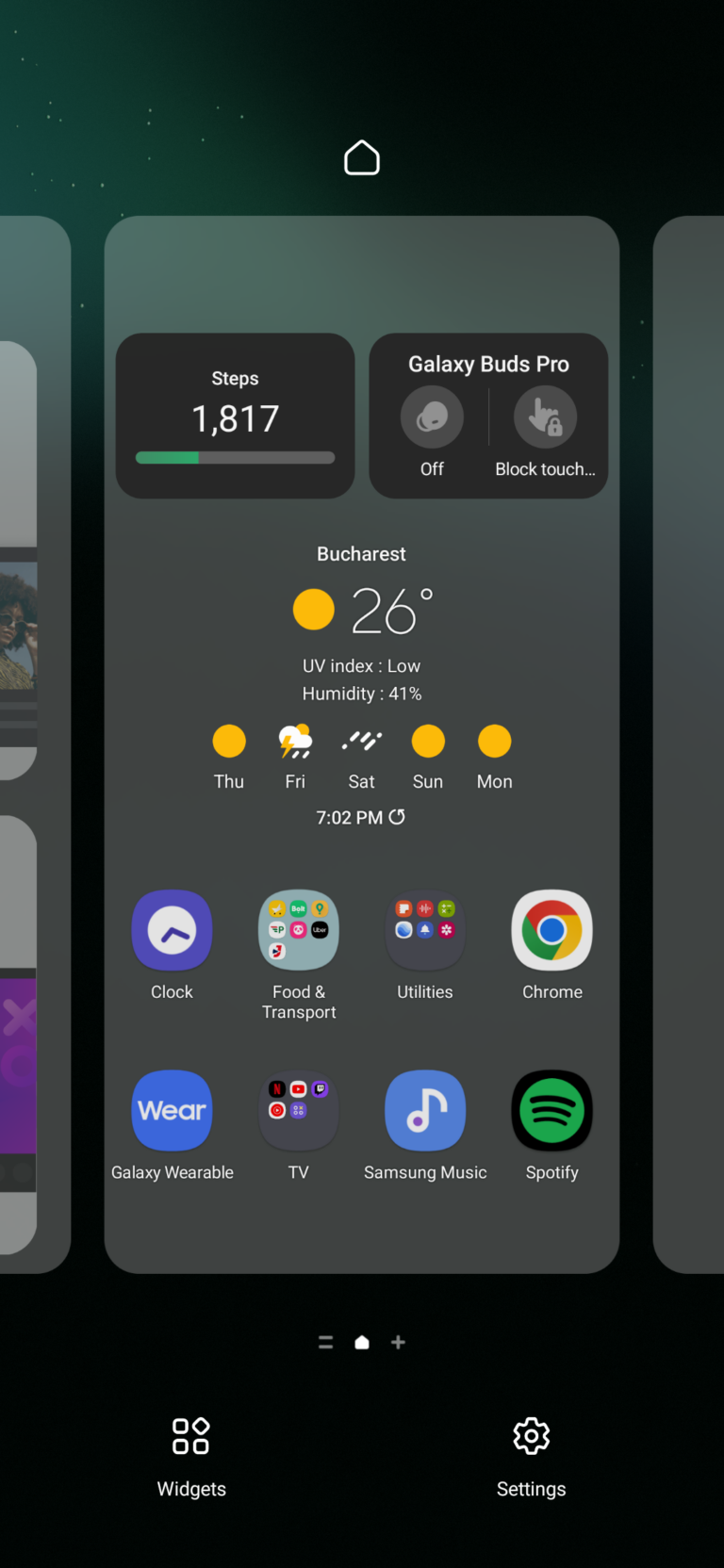This image captures a screenshot from a smartphone displaying multiple app interfaces and notifications on its home screen. At the center, the screen shows a step counter with a total of 1,817 steps, depicted by a partially filled gray bar with a green line marking the progress. At the top, there are two black rectangles; the first reads "Galaxy Buds Pro" indicating that the earbuds are off, and the second reads "black touch..." (implying an incomplete or cut-off notification).

Above this, in a darker section, the white home button is prominently displayed. Below the step counter, the screen features weather details under the heading "Butcher Rest." The current temperature is shown as 26°C with a small sun icon, alongside additional information including a low UV index and 41% humidity. Weather forecasts for the upcoming days are depicted through icons: Thursday's sun, Friday's lightning and storms, Saturday's rain, followed by Sunday and Monday with sun icons.

The time displayed at the top is 7:02 p.m., alongside a refresh option. Further down, the screen shows app icons for a clock, food and transport, utilities, Chrome browser, and at the bottom row, icons labeled Galaxy Wearable, TV, Samsung Music, and Spotify.